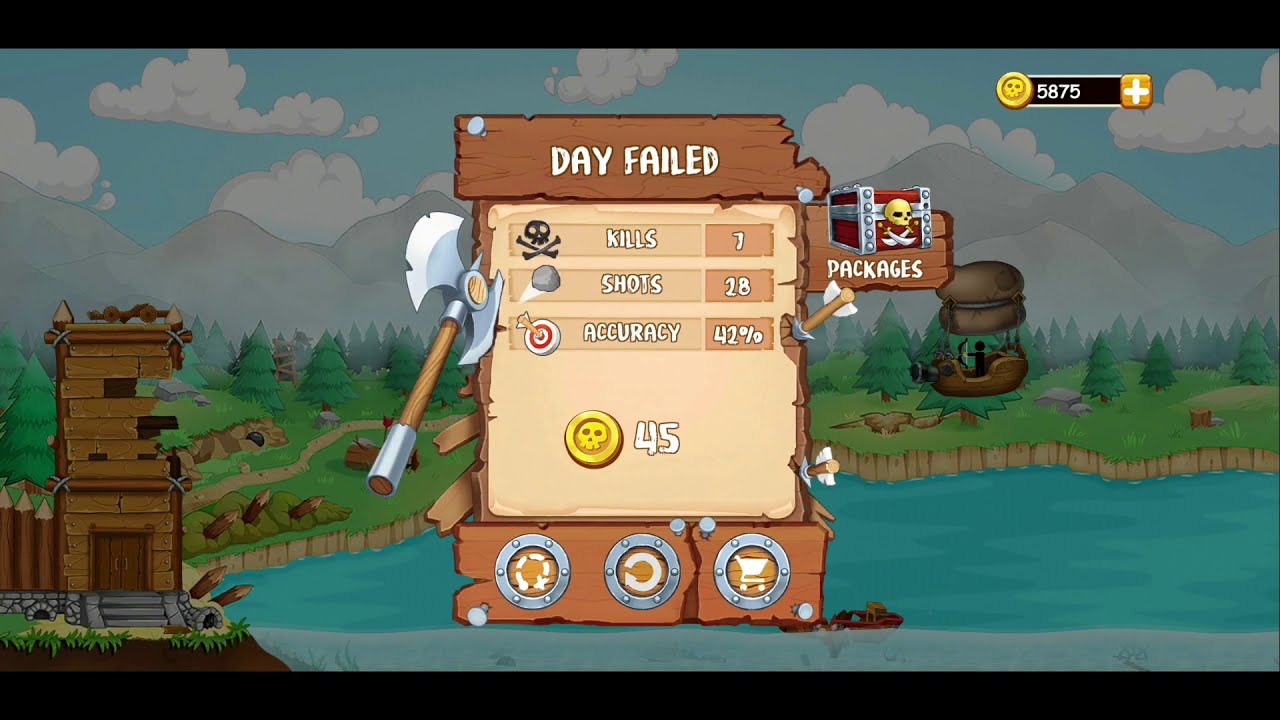The image depicts a screenshot from a cartoonish, animated video game. The scene is set outdoors with a variety of detailed elements. In the center of the image, there is a large pop-up screen displaying game statistics, which include the message "Day Failed" in white font at the top. Below this, the screen details the player's performance with icons and text showing "Kills: 7," "Shots: 28," and "Accuracy: 42%." Additionally, it features a gold coin icon with the number "45" next to it, likely indicating the player's collected coins. 

The screen itself has a paper-like appearance with some tears along the edges, and a gray skull icon adds to the aesthetic. On the left side of the screen, there is an 'X' button, and on the right, it mentions "packages" that can potentially be opened for new weapons.

The backdrop presents a scenic landscape, including a blue lake bordered by green grass, a line of trees, and gray mountains with clouds in the sky. In the bottom left corner, there's a disheveled wooden fort with stone steps, giving the impression of a somewhat dilapidated structure. Additionally, to the right of the main pop-up screen, a small black silhouette is depicted, riding a blimp with a bow in hand. The colors are vibrant, with the main pop-up screen in brown, tan, and silver hues, and the treasure chest on this screen is accented with red and silver, alongside gold elements indicating coin count.

Overall, the image combines detailed visual elements and game statistics to immerse players in the interactive, outdoor video game environment.